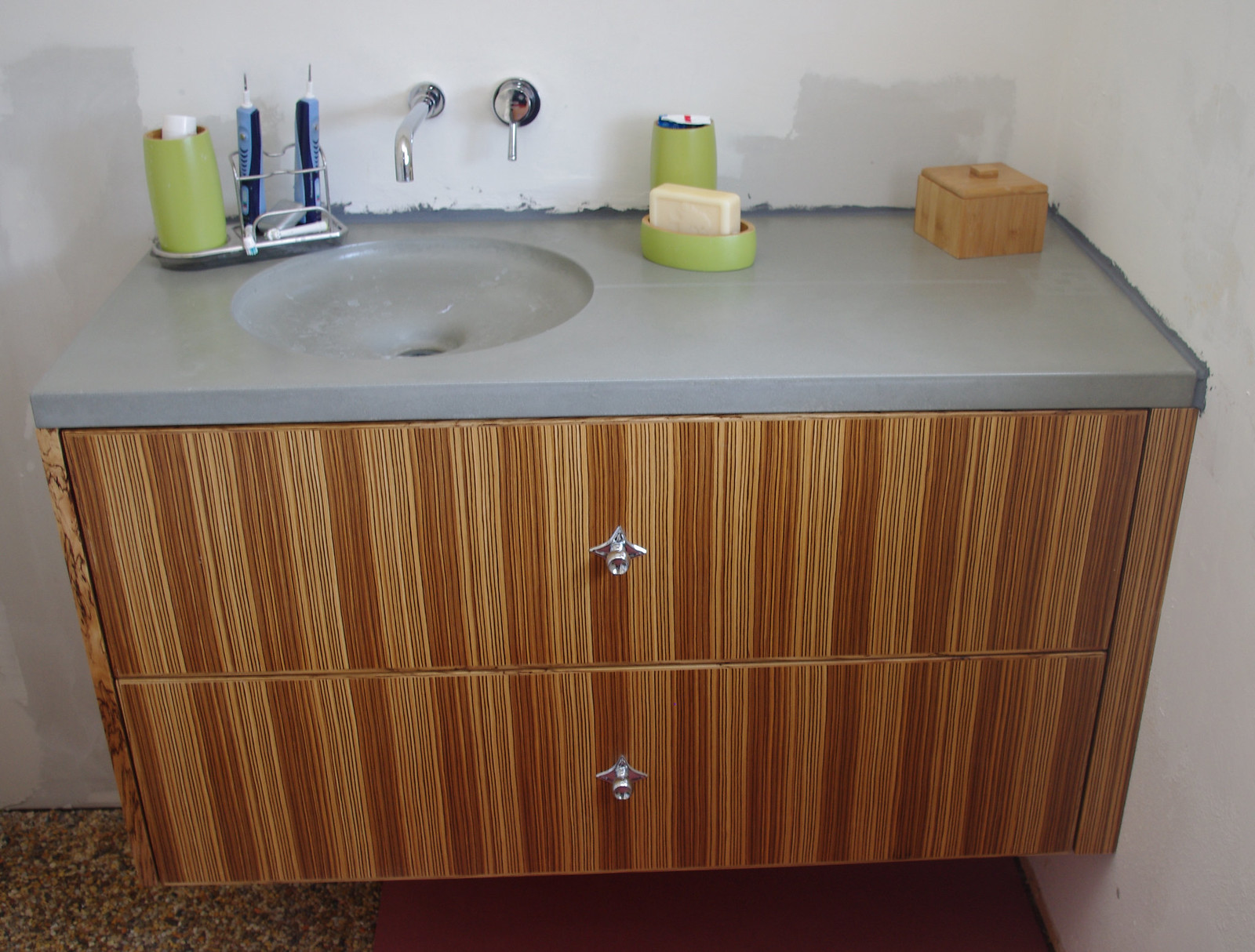The image showcases a detailed view of a bathroom sink area. The bathroom vanity features two drawers, with one positioned above the other. To the left, there is a sleek sink embedded in the vanity, topped with a gray countertop. On the countertop, to the right of the sink, there are several items arranged neatly: a set of green glasses, a green soap dispenser containing liquid soap, and a bar of soap. On the left side of the sink, a green container houses toothpaste and electric toothbrushes.

The sink itself has a modern faucet that extends directly from the wall, complemented by a push-button valve also mounted on the wall. Notably, the insulation around the faucet has been caulked, although the caulking job appears rushed and is characterized by jagged, messy lines.

Further to the right of the sink, there is a small container with a wooden handle on top, adding a touch of rustic charm to the contemporary setting. The bathroom's walls are painted a crisp white, providing a clean and bright backdrop. Interestingly, there is no mirror visible in the image, emphasizing the minimalistic and functional design of the space.